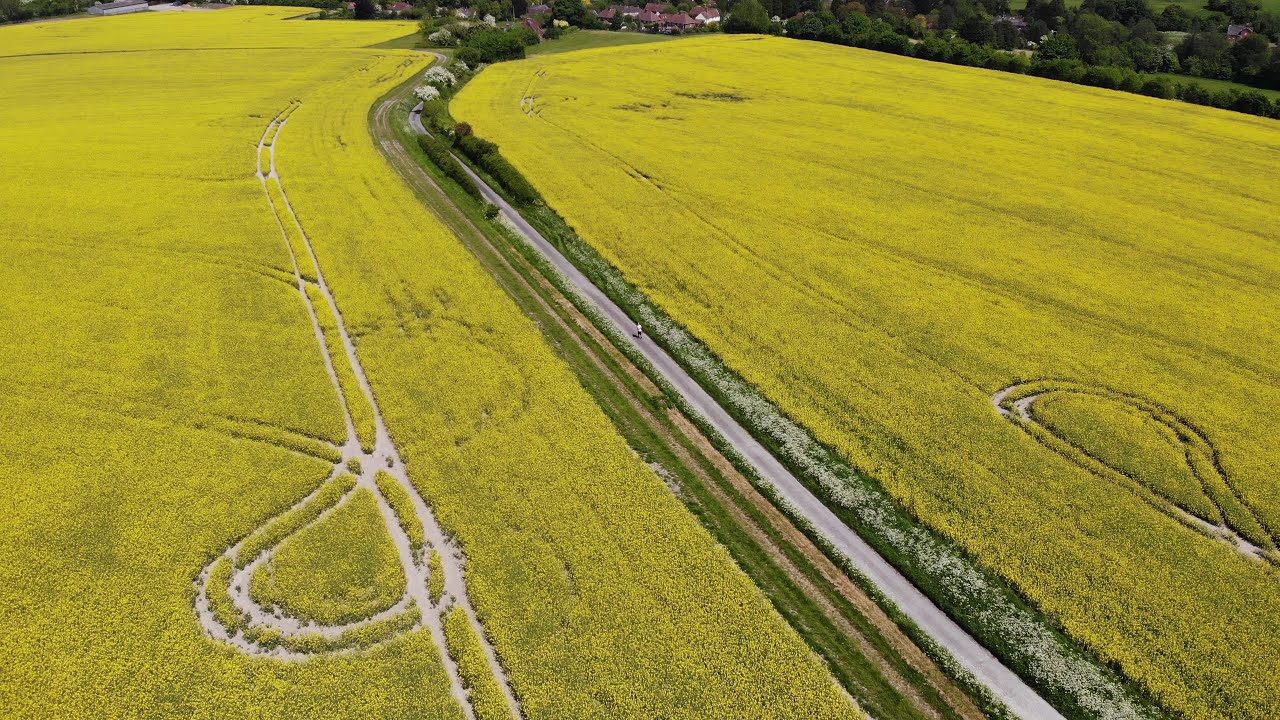This is an aerial daytime photograph capturing a vast agricultural landscape dominated by vibrant yellow fields, presumably filled with yellow-flowering crops. Bisecting the image from the lower right corner to the center top, before curving rightward, is a narrow, single-lane gray road. A small human figure, donned in a light-colored top and dark pants, is seen walking along this road, emphasizing the scale and vastness of the fields. Flanking both sides of the road are lush green strips adorned with white flowers, gradually transitioning into denser, hedge-like vegetation towards the top of the image. The fields themselves are intricately patterned with a mix of straight and curved vehicle tracks. In the upper right corner of the image, tall trees and a cluster of buildings with red roofs hint at a nearby village, adding an element of human habitation to this picturesque countryside.